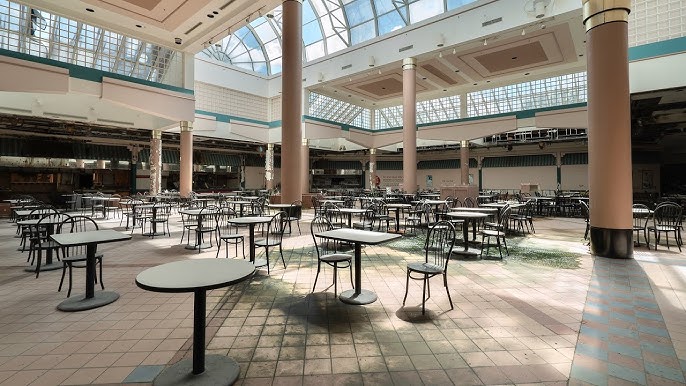The image depicts a spacious interior area that resembles either a cafeteria or a food court, possibly within a mall, an office building, or a school. The room is expansive and features a variety of small tables, both round and rectangular, each paired with black metal or hard chairs. The room is currently unoccupied, lending an air of stillness. 

The floors are tiled in a pattern of square shapes, alternating between shades of brown, blue, and a hint of pink. The ceiling is grand and filled with arched windows, allowing ample light to flood the space. The windows either offer a view of the sky, showcasing blue and white hues, or are painted to mimic this effect.

Large stone columns, painted in shades of brown with dark brown bases or possibly pinkish tones, are strategically placed throughout the room, extending from the floor to the high ceiling. These pillars add to the structural elegance of the space. An upstairs area is visible on the upper left, continuing across to the upper right, suggesting a multi-level design. The intricate details of the ceiling include a blue trim that complements the overall aesthetic of the space.